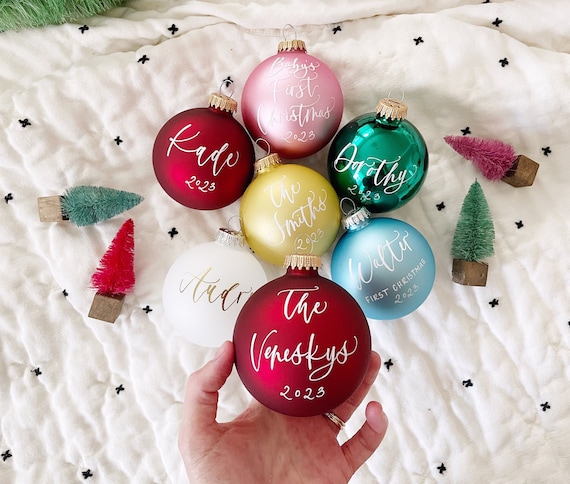Displayed on a soft, white blanket adorned with black crosses or X patterns is an array of festive, holiday-themed decorations. Scattered across the surface are miniature Christmas trees—two green, one red, and one pink—that are perfect for adorning a small dresser. Additionally, a collection of colorful Christmas balls enhances the holiday spirit, featuring two red, one pink, one yellow, one green, and one blue ornament. Each ball is detailed with white script, including inscriptions such as "K-2030" and "First Christmas 2003," although some of the text is faint and hard to read. The overall scene emanates a cozy, celebratory atmosphere.